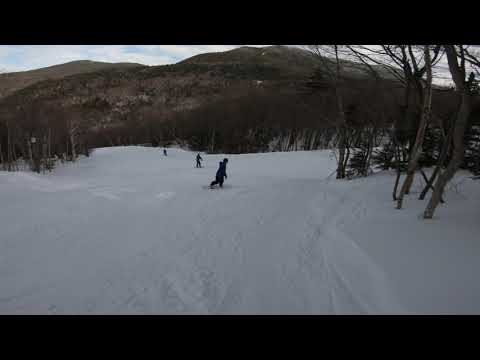An outdoor snowy landscape stretches into the distance, framed horizontally by long black bars at the top and bottom of the image. In the foreground, three people traverse the snow; the nearest is blurred and lacks detail, while the third is just a tiny speck against the expanse. Tracks mark their paths. The sky is mostly clear with a few clouds diffusing the sunlight, casting a dim light across the scene. To the right, a thin clump of barren trees stands, contrasting with the vast stretch of snow to the left. Dominating the background is a large, rocky mountain almost touching the top of the image, notable for its absence of snow and its brown hues punctuated by sparse green vegetation.